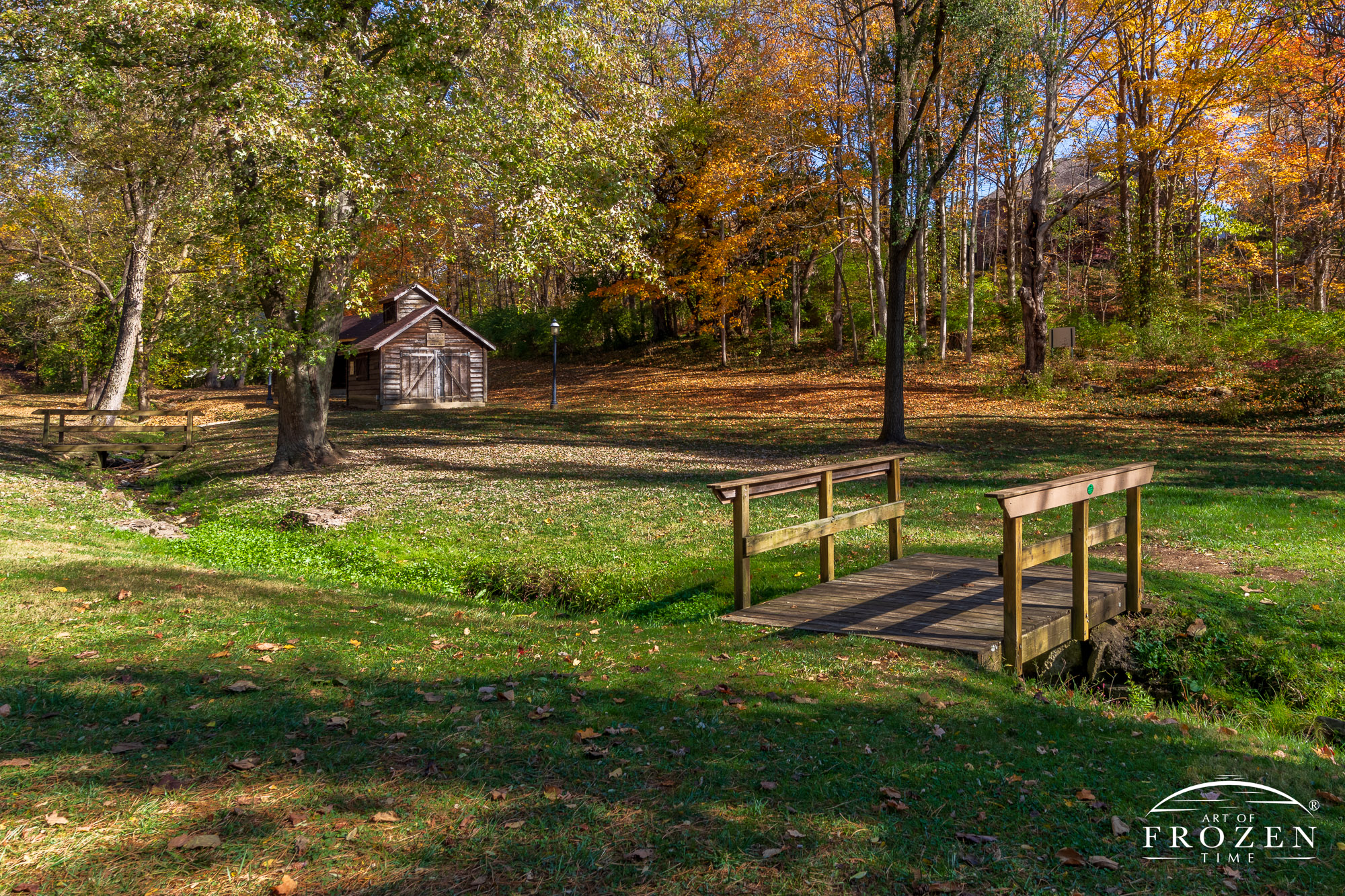This color photograph captures a serene, forested setting during the daytime, likely resembling someone's backyard retreat. A meticulously maintained grassy area dominates the scene, scattered with green foliage, white flowers, and the occasional dead leaf. Toward the right-hand side of the picture, a charming wooden bridge spans a small stream. The bridge, approximately 8 to 10 feet long and 6 feet wide, features two wooden railings, three support beams, and two side beams. In the background, a small log cabin-like house is visible on the left side, complemented by a nearby light pole that adds a quaint touch. Trees with autumn-colored leaves frame the image, creating a picturesque view. The text "Art of Frozen Time" is subtly inscribed in white lettering at the bottom right corner of the photograph.